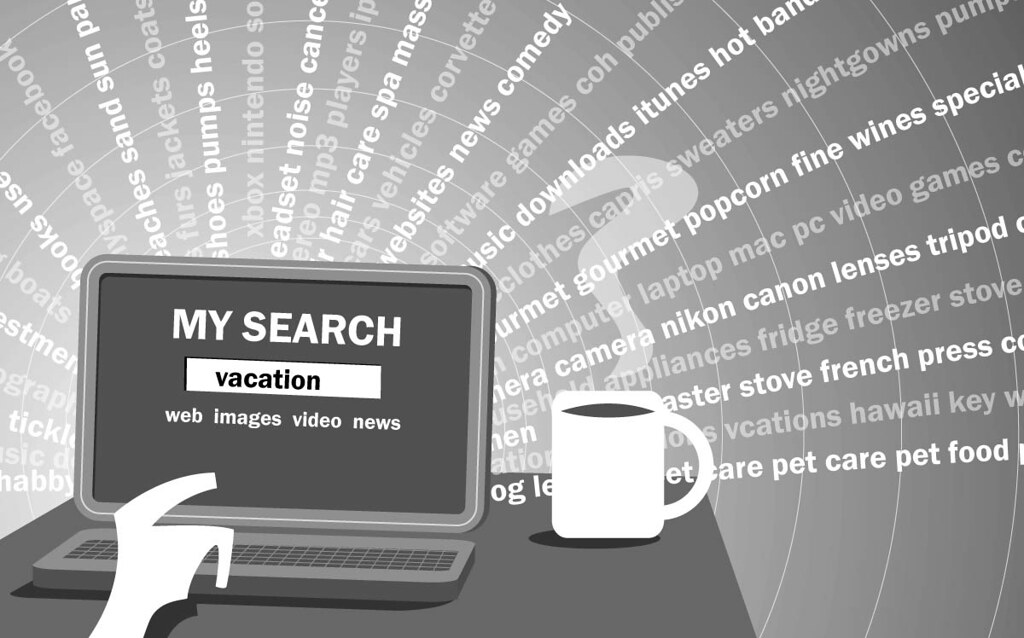The black-and-white computer graphic portrays a stylized scene of a desk with various items. Dominating the scene is a gray laptop or tablet on the left side of the dark desk. The screen prominently displays the term "MySearch" in all caps, followed by a search box containing the word "vacation." Beneath the search bar are tabs labeled "web," "images," "video," and "news." A white, cartoon-like hand with an outstretched finger appears poised to interact with the device.

On the right side of the desk sits a white coffee cup with steam curling up in a question mark shape, suggesting a freshly brewed beverage. Emanating from behind the laptop is a dynamic array of alternating white and gray words arranged in a sunburst pattern. These words—appearing to be potential search results or related terms—include "gourmet popcorn," "fine wine special," "computer laptop," "map," "PC," "video games," "camera," "Nikon," "Canon lenses," "tripod," "appliance," "fridge," "freezer," "news," "comedy," and "sweaters," among others.

Overall, the graphic combines various elements evocative of an online search experience, visually illustrated through the interplay of text and imagery.